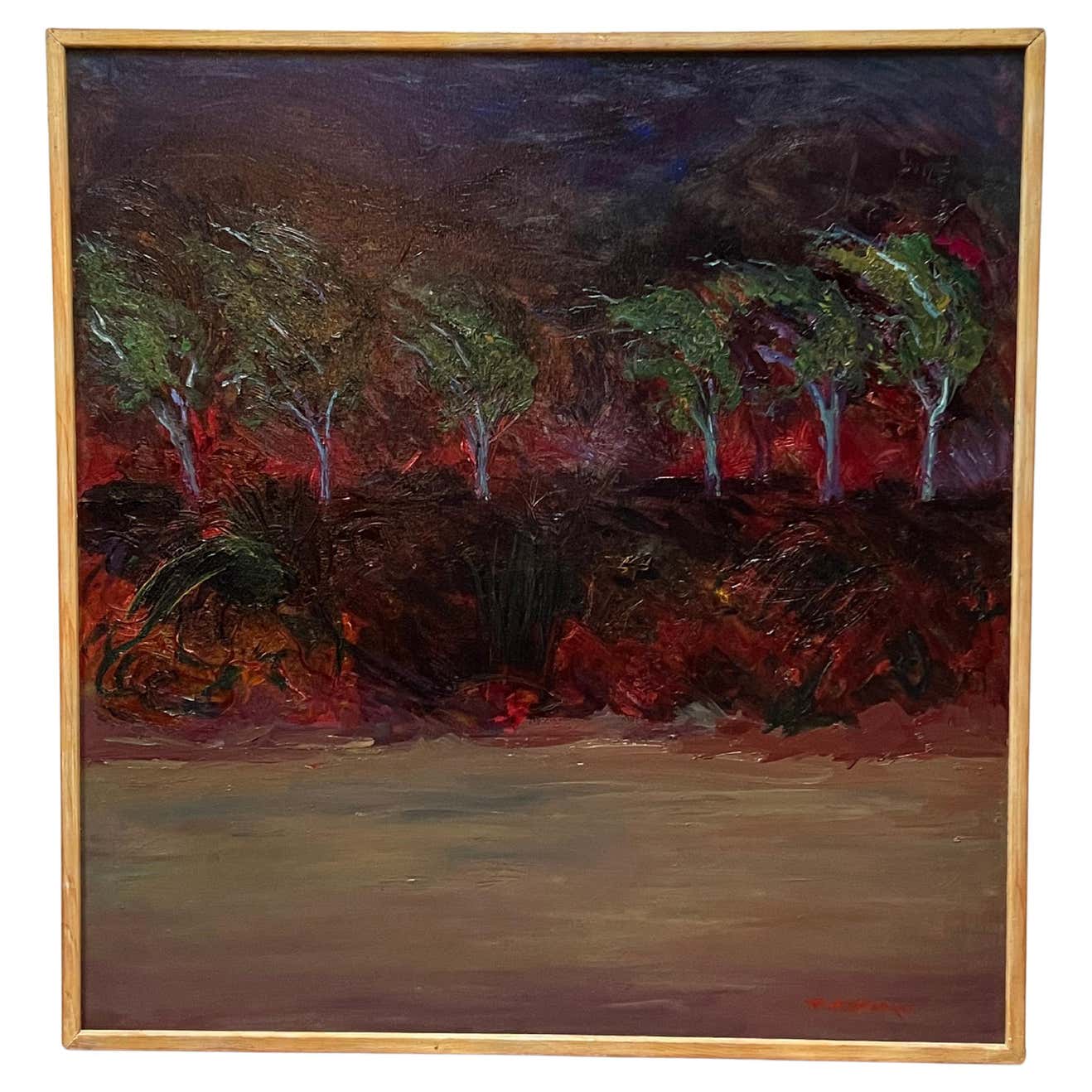The photograph captures a painting enclosed in a light brown wooden frame. The artwork, rendered in thick oil or acrylic paints with an impressionistic watercolor style, vividly depicts a natural scene characterized by tumult. At the base, there's a sandy area transitioning into a grassy, hilly terrain imbued with dark, reddish-black tones that evoke a sense of destruction, possibly from a wildfire. Atop this bank is a forest featuring six trees, their light gray trunks juxtaposed against splotchy green leaves that appear to be blowing in the wind. The riverbank itself displays a palette of aggressive colors, including dark green, brown, and bright red, with the water painted in murky shades of light green to gray. Above the trees, the night sky looms ominously with layers of black, dark blue, light purple, and brown, intensifying the scene’s dramatic and turbulent atmosphere.